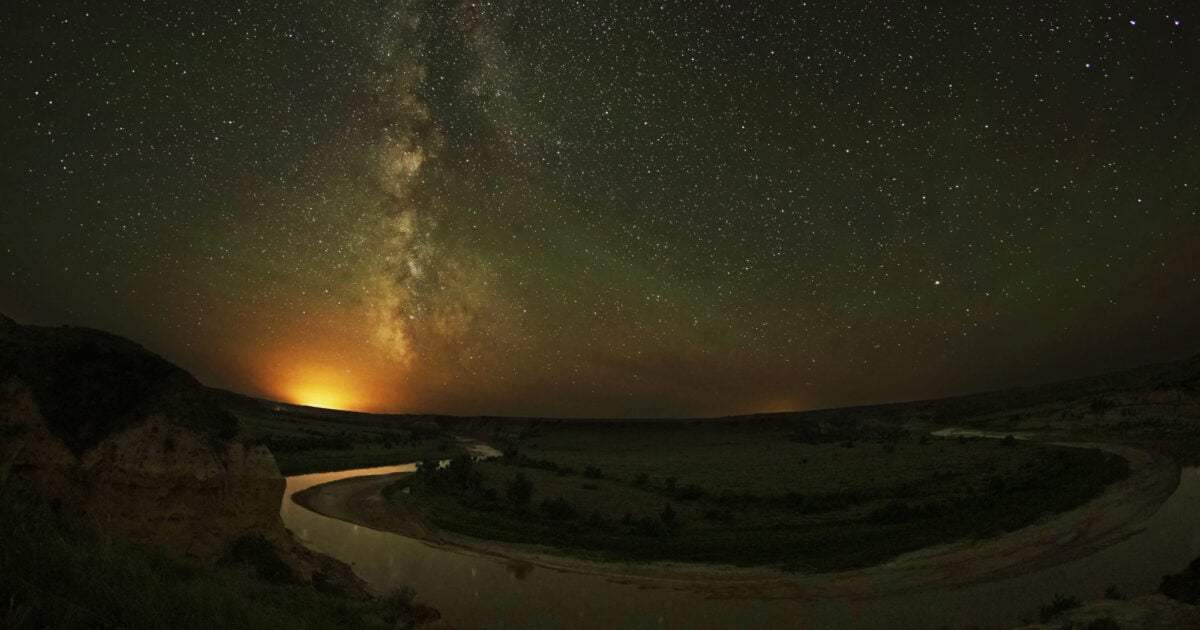This panoramic image captures a stunning night scene with a star-filled sky over a darkly silhouetted landscape. The sky, a darkish purple hue with tinges of green, orange, and blue, is adorned with a multitude of stars, some forming cloud-like swirls that stretch to the top of the frame. A bright light on the horizon, perhaps the last sliver of the setting sun, adds an additional glow to the twilight atmosphere. The land below is quite dark, obscuring clear details but suggesting the presence of grassy hills or mountains in the distance. A circular feature, possibly a moat around a man-made island, is faintly visible, with water trailing off into a creek or stream. A small rock formation in the foreground hints at the rugged nature of the terrain. It's ambiguous whether this highly detailed and serene nightscape is a photograph or an incredibly realistic drawing.